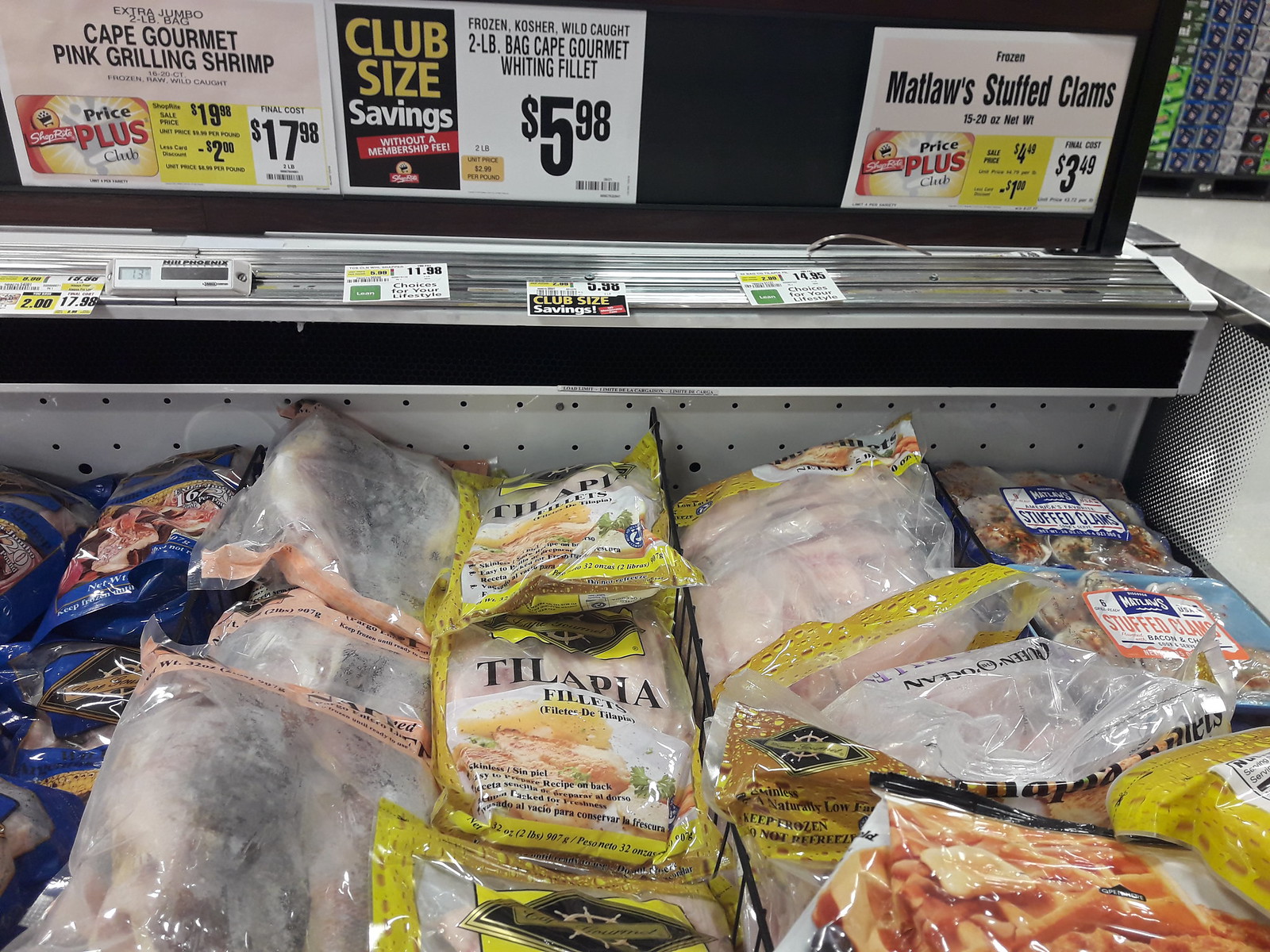The image displays a section inside a grocery store’s frozen food aisle, specifically showcasing a variety of pre-packaged seafood items. Positioned predominantly at the bottom of the image within the freezer are packages of Cape Gourmet Pink Grilling Shrimp, a 2-pound bag of Gourmet Whiting Filet, and Mass Loss Stuffed Clams. The seafood items are arranged with their respective price tags and signs just above them. 

The signs are placed within a black frame at the top of the freezer, detailing promotional prices for ShopRite Price Plus Club members. The sign on the left advertises the Cape Gourmet Pink Grilling Shrimp at a final cost of $17.98. The middle sign indicates a club size savings for the 2-pound bag of Cape Gourmet Whiting Fillet, priced at $5.98. On the right, the sign promotes frozen Matlaw Stuffed Clams for $3.49. 

The colors visible in the image include black, white, yellow, red, blue, and orange, reflecting the diverse packaging and promotional materials. The setting is clearly indoors, within the frozen food section of a supermarket, but the exact time of day remains indeterminate.